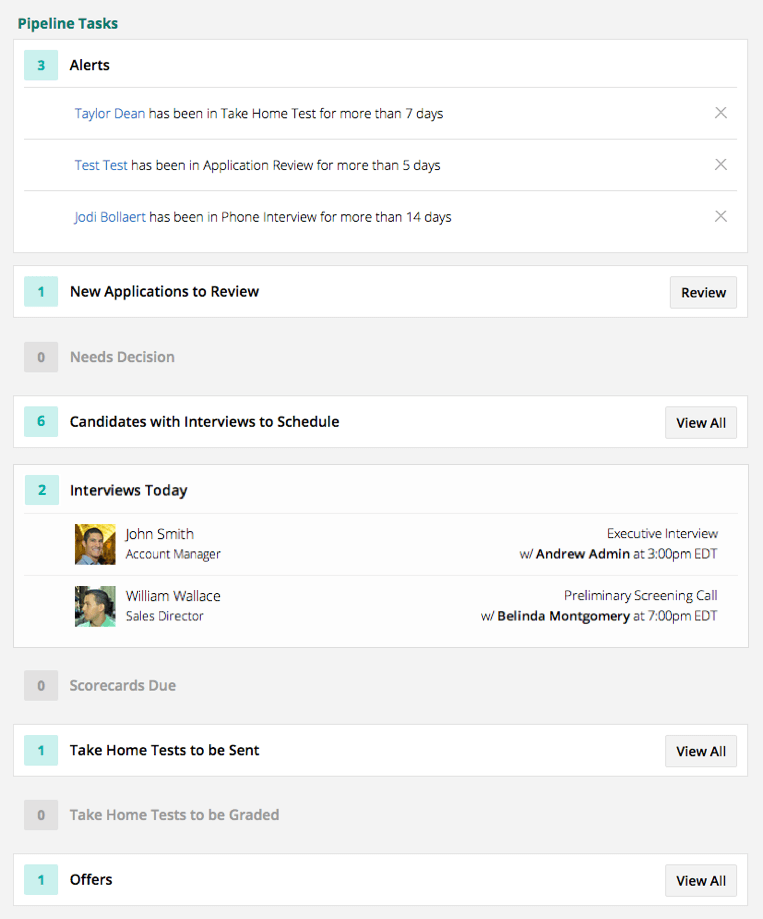The image is a screenshot of an employee management platform focusing on pipeline tasks. At the top, a heading reads "Pipeline Tasks" in prominent text. Below this, encased in a light green box with a darker blue array, is the number "3" signifying a section about alerts.

In this alert section:
- Taylor Dean is indicated in blue text, followed by a note in black text stating, "has been in take-home test for more than seven days."
- In the subsequent alert, "Test Test" appears in blue text, with black text noting, "has been in application review for more than five days."
- Another alert shows "Jody Bollert" in blue text, accompanied by black text stating, "has been in the phone interview stage for more than 14 days."

Proceeding this section:
- A light green box with a numeral "1" denotes "New Applications to Review" with a corresponding "Review" button on the right.
- Underneath, a gray box marked with the numeral "0" designates "Needs Decision."
- Further below, a light blue or green box enumerated with the numeral "6" represents "Candidates with Interviews to Schedule," along with an option to "View All."
- This is followed by a section in light blue or green text labeled "Interviews Today," listing:
  - John Smith, Account Manager, and
  - William Wallace, Sales Director, each with their respective thumbnail profile pictures.

Continuing below:
- A segment in gray text shows "0 Scorecards Due."
- The next sections offer buttons to "View All" for tasks such as:
  - "Take-home tests to be sent,"
  - "Take-home tests to be graded," and finally,
  - "Offers."

This detailed breakdown highlights various actionable items and statuses within the employee management tool, aiding users in prompt decision-making and task prioritization.